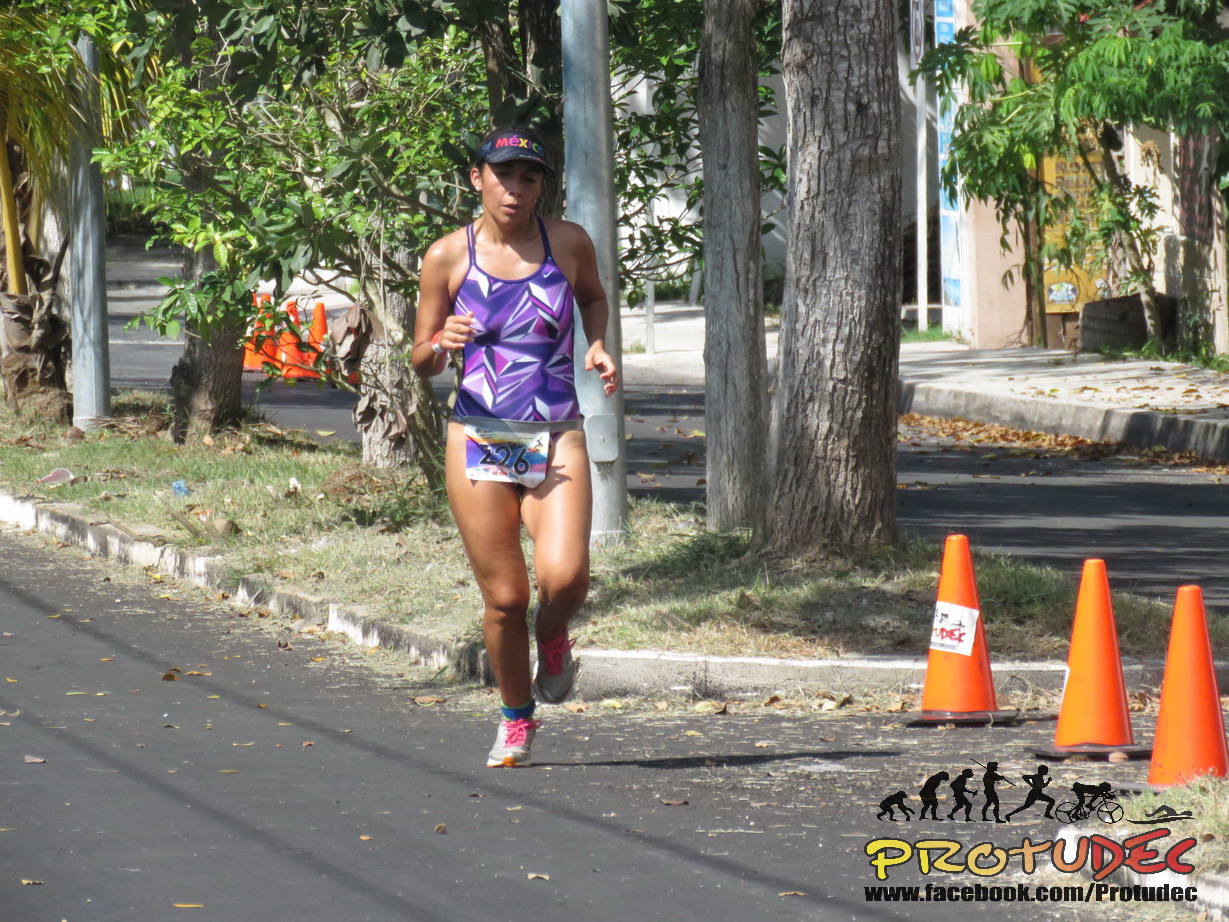A tanned marathon runner, wearing a black baseball cap with colorful designs that reads "Mexico," and sporting a purple and pink patterned tank top, dashes down a city street. She is wearing very short shorts and has pinned to her front the race number 226. Her feet are adorned with white running shoes featuring bright pink laces. The race route is lined with trees, grass medians, and several light fixture poles. Behind her are brick buildings, possibly city structures or a parking ramp. Three orange safety cones block off a side road to her right. At the bottom right corner of the image, text reads "Pro2Deck, www.facebook.com/Pro2Deck."